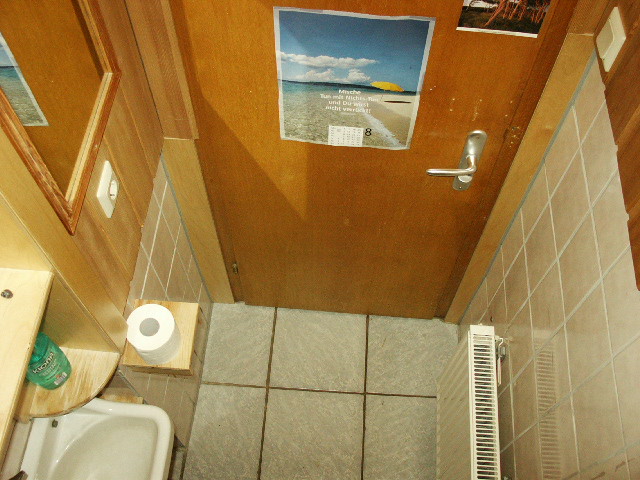This aerial view of a bathroom reveals a detailed layout with various objects and fixtures. Dominating the center background is a wooden door with a silver handle and a lock at the bottom. Attached to the middle of the door is a poster featuring an image of a road, with small, unreadable text. Another partially visible poster is located at the top right of the door, alongside a light switch. To the left of the door is a wall-mounted mirror with a wooden frame, adjacent to a porcelain white sink. The sink is accompanied by a wooden ledge holding soap, and a separate wooden ledge to the right displays a roll of toilet paper. The entire space is tiled with white tiles on both the floor and walls. Additional details include a radiator positioned next to the door and a hint of a bottle of mouthwash near the sink. The color palette of the bathroom encompasses yellow, blue, tan, white, green, black, red, and brown hues, creating a coherent yet vibrant setting.